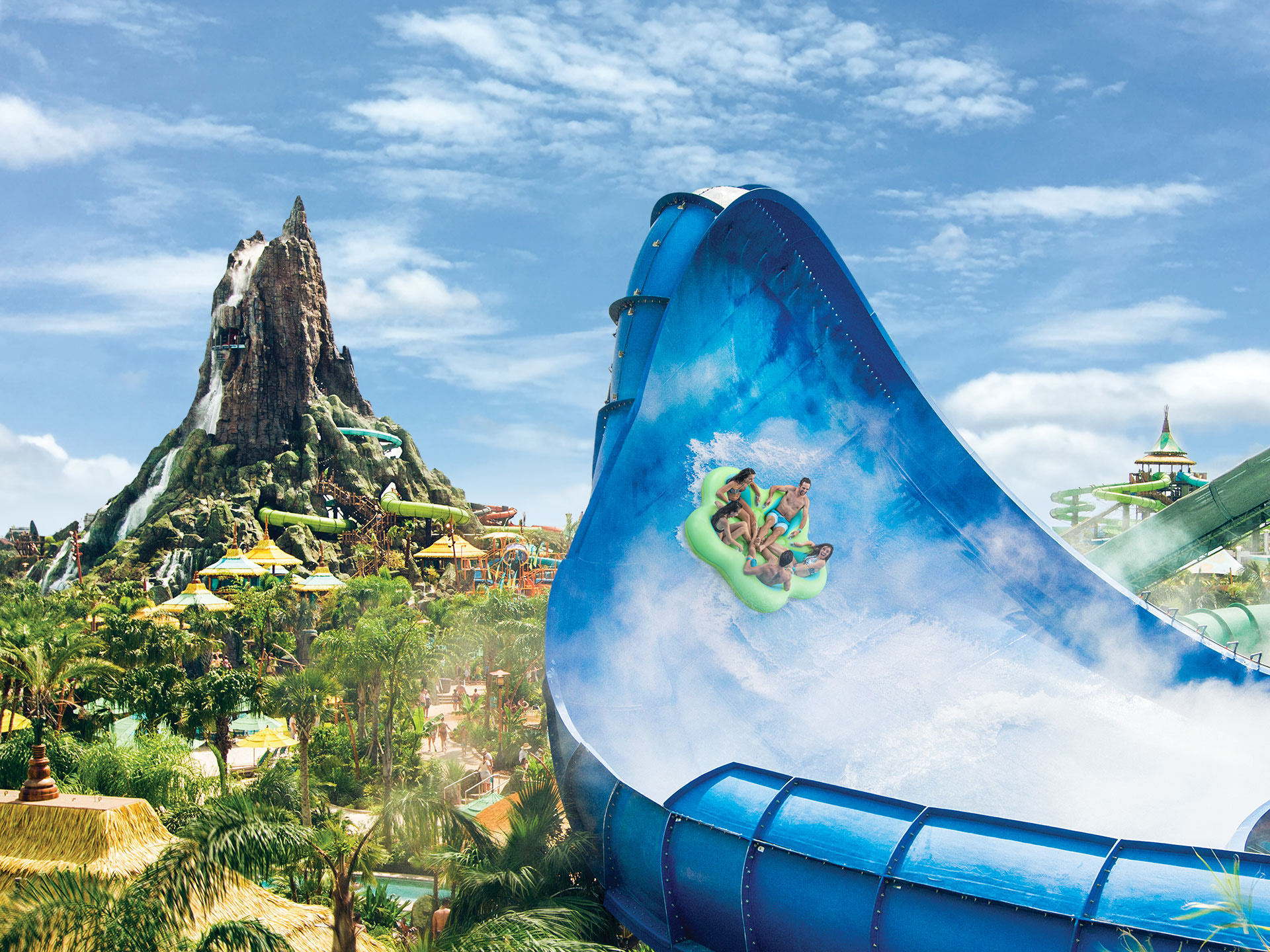The image depicts an artist's conception of a photorealistic water park set in a jungle-like environment. Central to the scene is a large, winding blue water slide that towers skyward before descending into a white-blue waterway. Midway down the slide is a lime-green inflatable raft carrying a family of five—two adults and three children—all in bathing suits, lounging and enjoying the ride. The sky above is a clear blue, dotted with fluffy white clouds. 

To the right stands a tall mountain, integrated into the water park with slides of yellow and blue tubing weaving in and out of its structure. A waterfall cascades from the mountain's peak, adding to the idyllic setting. Adjacent to this, another attraction features a green tube leading to a pointed trellis or pavilion, from which multiple slides emanate.

The left side of the image is lush with varied vegetation, including palm trees, ferns, and other trees, some planted in wooden vases that sit on yellow, hay-like platforms. Straw-roofed huts and yellow-green umbrellas add to the rustic charm, while a makeshift river, possibly a lazy river, flows gently at ground level. This immersive scene captures the essence of a tropical paradise, blending natural elements with the thrills of a water park adventure.